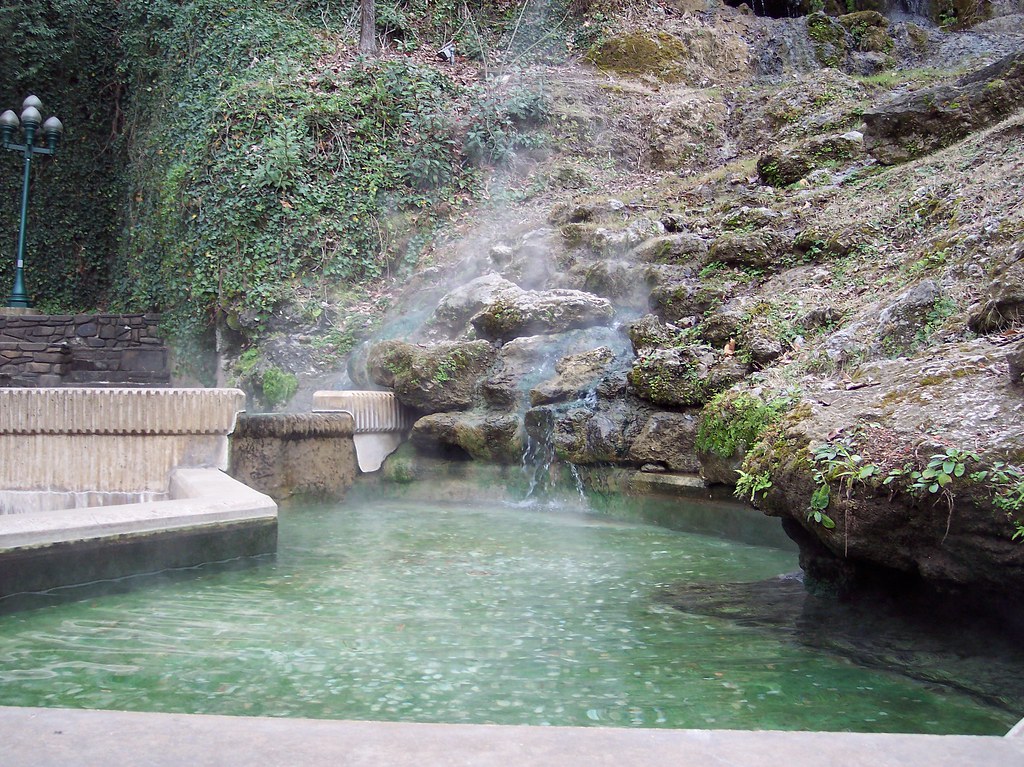This color photograph captures a serene, possibly artificial, hot spring. A small, trickling waterfall descends over a mossy, vine-covered rock outcropping at the back of the image, releasing steam into the air. The waterfall flows into an irregularly shaped pool with rounded edges, filled with green-tinged water. The pool is bordered by a concrete base. On the left side of the image, there is a stone wall and white sitting areas, as well as a green lamppost in the upper corner. To the right, the pool merges with lush green fauna and an upward-extending hill. No people, animals, or vehicles are visible, contributing to the peaceful ambiance of the scene.